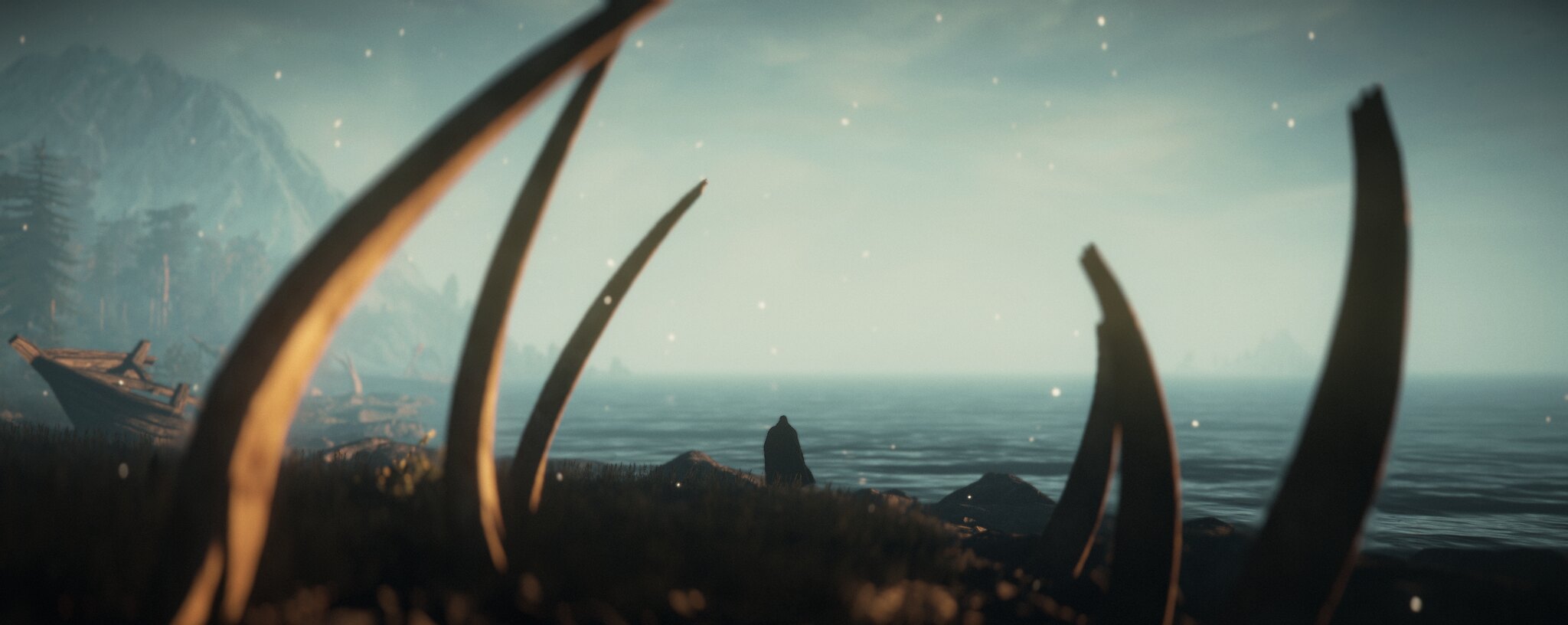The image is a highly detailed landscape-oriented illustration, possibly from an animated film or a game. The scene is set on a shadowed shoreline, low to the ground, with realistic water in the background showing ripples from either waves lapping or wind blowing. In the foreground, large, ribcage-like structures or the remnants of a broken boat curve upwards, encircling the camera and extending into the distance. To the left, near the bottom third of the image, a weathered wooden boat sits on the shore. Further back and to the left, hazy mountains rise out of the frame, with misty pine trees nearby. The horizon features a foggy white sky that obscures most of the background, while streaks of bluish sky peek through in the top right, casting a cold, wintery tone over the scene. Rocky and grassy areas with scattered boat debris and dark, shaded patches complete the rugged, desolate atmosphere of the artwork.